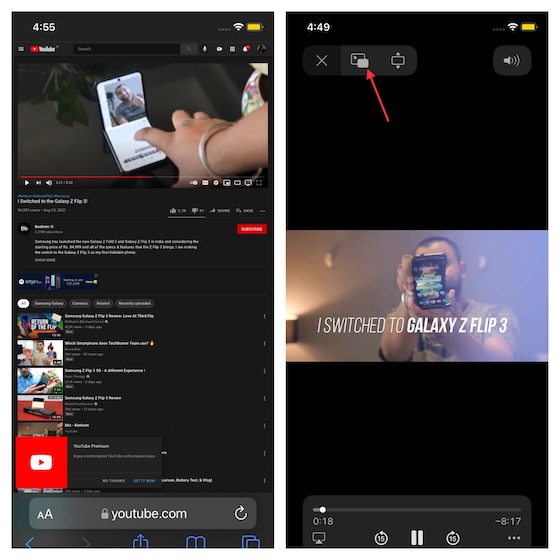A detailed caption for the image based on the provided description:

"A person on the left side of the image is looking at a smartphone, specifically a flip phone, which displays '455' on its screen. The scene transitions to a YouTube interface, highlighting a standing phone being tapped. The phone model is identified as the Galaxy Z Flip 3, shown in the center of the image with the screen slightly folded, displaying a 'Subscribe' button alongside various multimedia elements such as pictures, text, images, and videos. The YouTube interface also indicates YouTube Premium at the bottom left, with icons for YouTube.com, left arrow, right arrow, open book, and two square shapes. To the right, the screen displays '449', along with full Wi-Fi, full battery status, and an 'X' icon. Additional interface controls include a speaker icon and a mostly black background. At the center, the phrase 'I switched to the Galaxy Z Flip 3' is visible alongside someone holding the folded phone. The video is at the 18-second mark, with 8 minutes and 17 seconds remaining. There are playback controls such as an AirPlay icon with a square and triangle, a 'reverse 15 seconds' button, a 'pause' button, a 'forward 15 seconds' button, and an ellipsis (dot, dot, dot). The top of the image contains some unspecified elements."